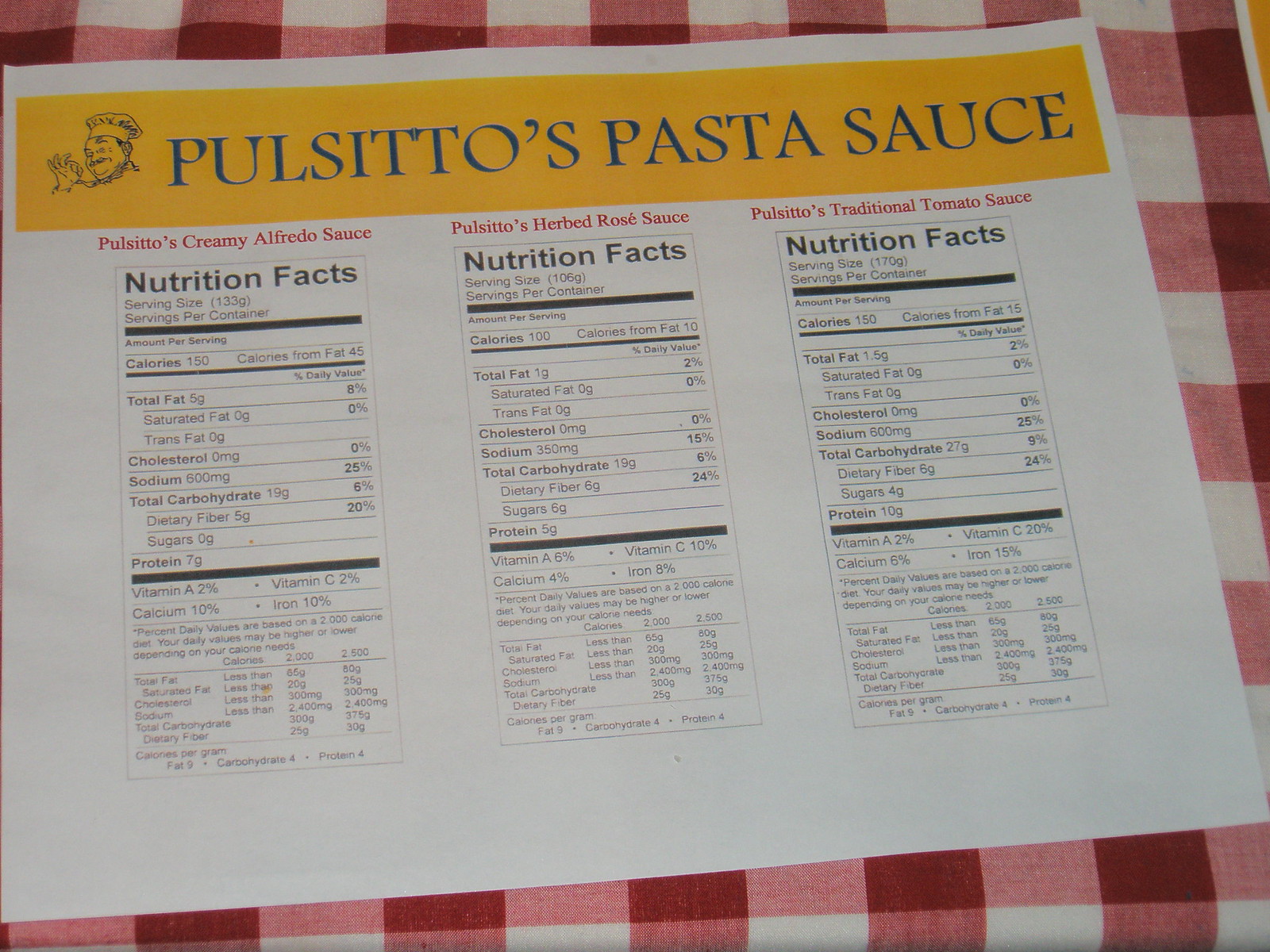The image features a piece of paper displaying nutrition facts for various Pulsatitos pasta sauces atop a red and white plaid tablecloth. At the top of the paper, an illustration of an Italian man making a traditional hand gesture is shown, complete with a chef's hat. The paper is divided into three sections, each dedicated to a different Pulsatitos sauce: 

- On the left is Pulsatitos Creamy Alfredo Sauce, 
- In the middle is Pulsatitos Herb Rosé Sauce,
- On the right is Pulsatitos Traditional Tomato Sauce.

Each section details the specific nutrition information for its respective sauce. The serving sizes differ for each: the Creamy Alfredo Sauce has a serving size of 133 grams, the Herb Rosé Sauce is 106 grams, and the Traditional Tomato Sauce is 107 grams. Notably, the Traditional Tomato Sauce offers a slightly larger serving size compared to the other two, making it the most abundant in terms of quantity per serving.